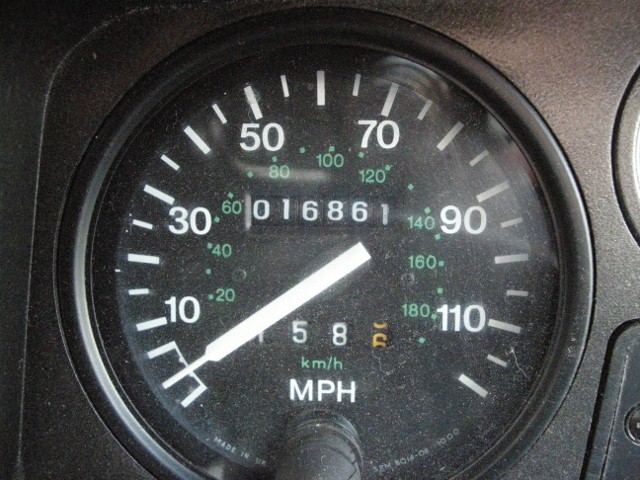This photograph captures a close-up view of a vehicle's speedometer set against a black dashboard. The dominant feature is the large, white numerals indicating speed in miles per hour, marked at 10, 30, 50, 70, 90, and 110. In contrast, the secondary speed markings in kilometers per hour are shown in a smaller, green font at intervals of 20, 40, 60, 80, 100, 120, 140, 160, and 180. 

The speedometer is encircled by a sleek black ring, enhancing its readability. Below the speed markings, the odometer displays the mileage as 016861, with the trip meter reading 158 miles. A small knob situated at the center of the gauge is used to reset the trip meter. 

Additionally, parts of adjacent dashboard gauges are partially visible, though their specific functions remain unclear. The size difference between the miles-per-hour and kilometers-per-hour fonts is notable, with the former being over three times larger, emphasizing its prominence. The green hue of the kilometer markings suggests they may offer enhanced visibility, potentially glowing in the dark for nighttime readability.